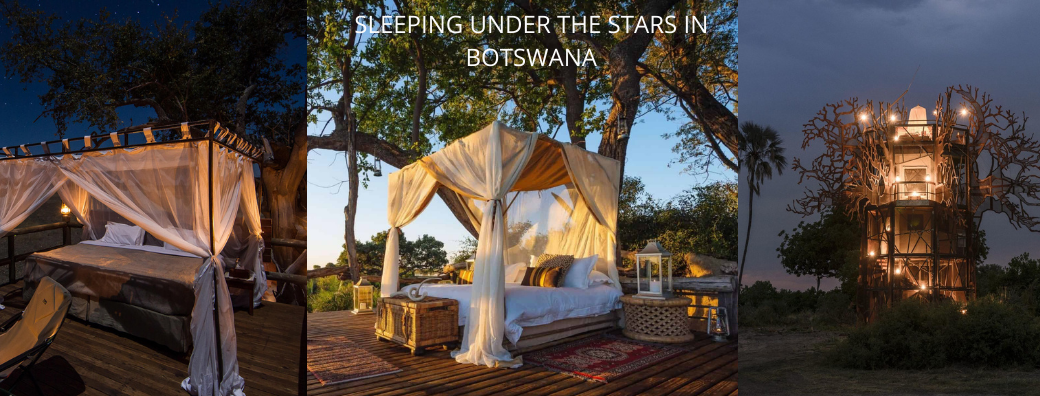The image is a collage of three photographs advertising an outdoor environment titled "Sleeping Under the Stars in Botswana," written in white text in the center. The left section shows an outdoor bed with white netting draped over a brown mattress, accompanied by white pillows. The bed is nestled beneath a dark green tree, and the mosquito nets are open at the front, tied to the posts, all set against a backdrop of a dark night sky. The middle section features a similar outdoor bed with a white mattress and mosquito nets that are a mix of darker white and brown. These nets cover the back but are open on the sides and front. The bed rests on a wooden floor made of 2x4s, and a round table with a lattice pattern stands beside it. Tall green trees rise above the scene. The right section of the collage depicts a unique, three-level treehouse, adorned with white lights and orange hues, enhancing its visibility against the dark, cloudy night sky. A palm tree stands just to the left of this illuminated structure.